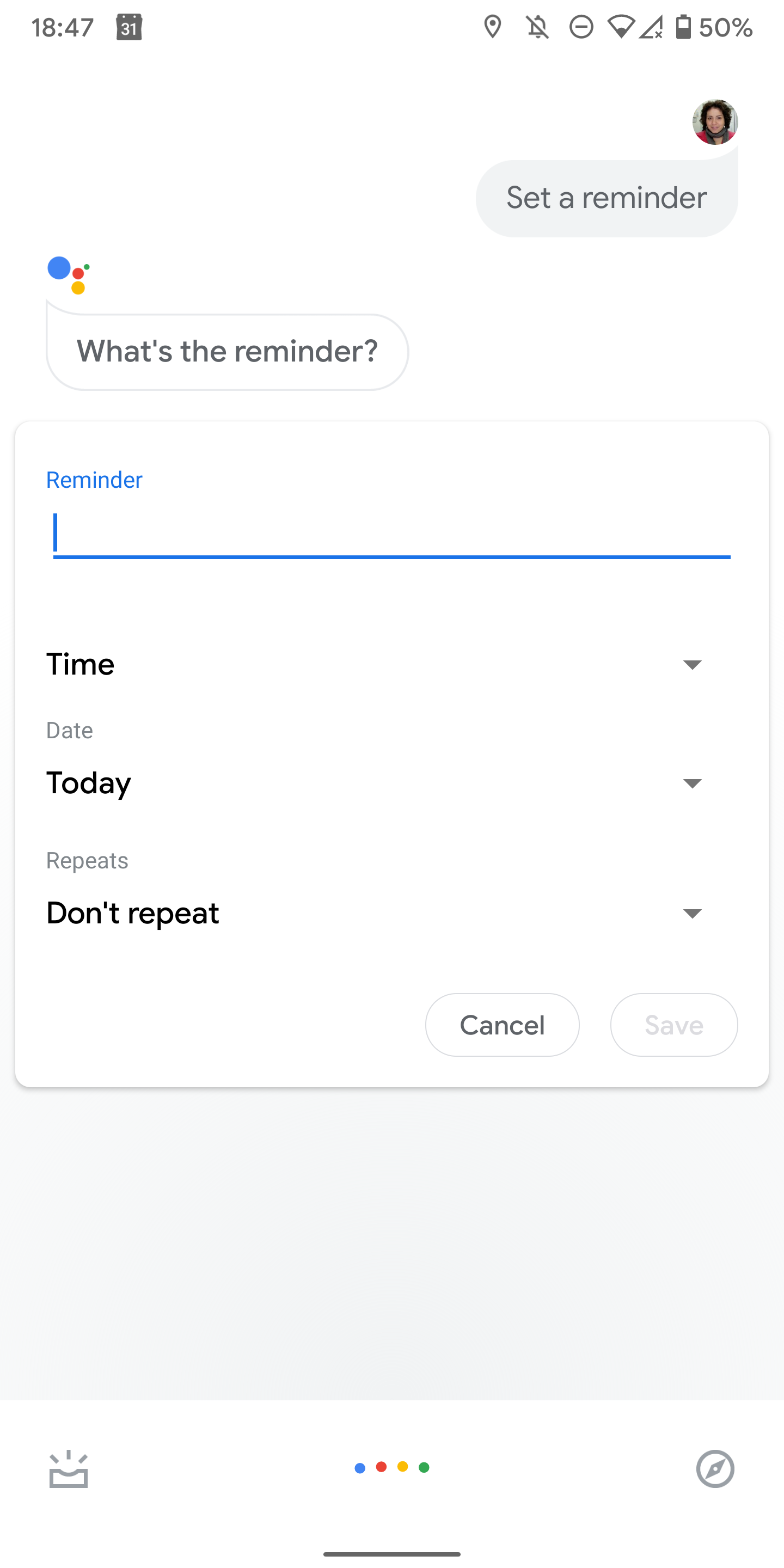This is a screenshot of a smartphone screen displaying the interface used to set a reminder. The background is predominantly white, and the time "18:47" is shown in black text in the top left corner. To the right, there is a black square icon representing a calendar with a white "31" inside it. Adjacent to this, the phone's status icons are displayed: a battery icon indicating it is 50% charged, an internet icon with an "X" showing the Wi-Fi is turned off, and a sound icon showing the sound is muted. The location icon is on, shown slightly to the right of the sound icon.

Below these icons, on the right side, there is a profile picture of a woman with short hair, wearing a black scarf and a red shirt, with a white wall in the background. Beneath her profile picture, there is a gray speech bubble containing the text "Set a reminder" in black. 

To the left of the bubble, there are multiple colored circles: a blue circle at the top, followed by a small red circle, a yellow circle beneath it, and another white speech bubble containing the text "What's the reminder?" in black.

Further down, there is a white square. Inside the square, "Reminder" is written in blue at the top left, followed by a blue line. Below this, "Time" is written on the left side with a dropdown icon on the right. Under that, "Date" is written in small black text, followed by "Today" in bold, with a dropdown arrow next to it. Below this, "Don’t repeat" is displayed in bold with another dropdown arrow to its right. "Save" and "Cancel" tabs are located in the bottom right corner of this section, with the "Save" tab in gray lettering and the "Cancel" tab in black. The entire section is bordered by a light blue line at the bottom, and the bottom inch of the screen has a white border.